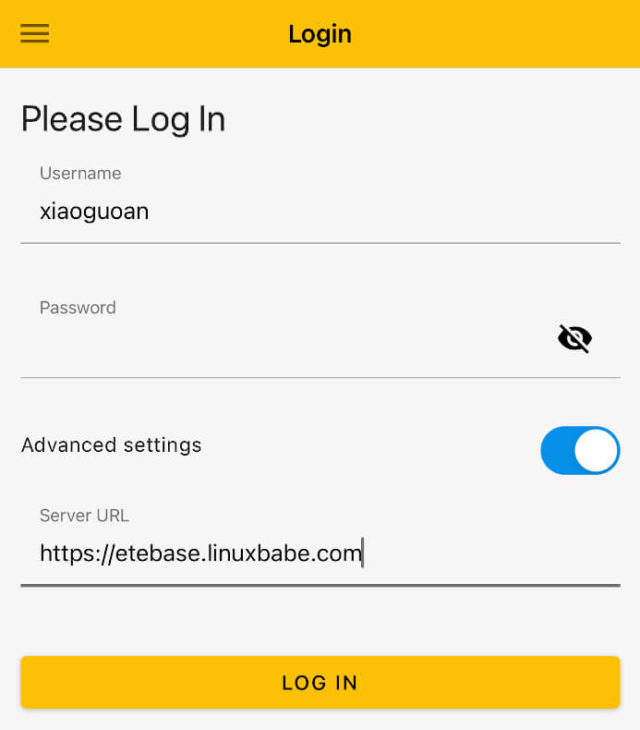**Caption:**

The image showcases a screenshot of a login interface for an unspecified app. The top section of the screenshot features a yellow background with the word "login" prominently displayed in the center using a black font. To the right of the "login" text, three horizontal black lines (representing a menu) are visible.

Beneath this yellow header, the rest of the interface is primarily gray. At the top of this gray section, it reads "Please log in." Below this prompt, there is a field for the username, pre-filled with the text "XIAOGUOAN". The password field is empty and is accompanied by the standard eye icon with a line through it, indicating the option to show or hide the password.

Further down, on the left side, there's an option labeled "Advanced settings." The icons associated with these settings are aligned to the right of the text. One notable feature within this section is a blue and white toggle switch, currently in the "on" position, likely for enabling or disabling specific advanced options. The field for the server URL is also present, showing an address that starts with "HTTPS."

At the bottom of the interface, there is a prominent yellow button labeled "Login," inviting users to proceed with the authentication process.